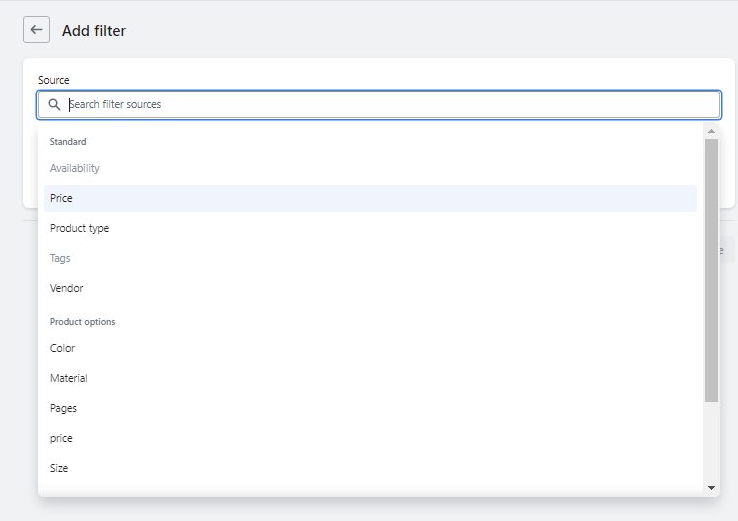This image depicts a detailed view of a search interface on what appears to be a sales or inventory management website. At the very top, there's a gray and tan navigation bar, featuring a black text option labeled "Add Filter" accompanied by a left-pointing arrow. Below this, there's a prominent white search box with black lettering indicating "Source." Adjacent to this box is a small spyglass icon, further labeled with the black text, "Search Filter Sources." 

Directly beneath this search area is a comprehensive list of searchable categories, all in black text. These include "Standard," "Availability," "Price," "Product Type," "Tags," "Vendor," "Product Options," "Color," "Material," "Pages," "Price," and "Size." Users can scroll down through these options to refine their searches. Underneath this list lies another gray and tan box, presenting various selections for filtering search results.

The layout and options suggest that this interface is part of a robust software solution designed for managing inventory or sales. Users can filter through diverse criteria such as price, product type, vendor, and material to efficiently search their inventory.